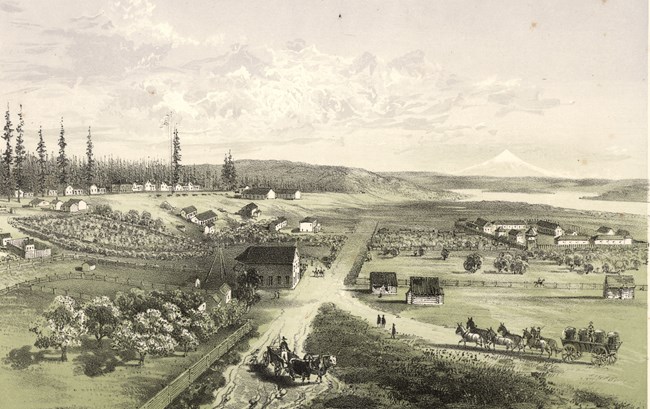This sepia-toned artwork, resembling a black and white photograph, offers an intricate aerial view of a historic settlement, likely from the mid-1800s in the United States. The scene is dominated by a wide dirt road running through the center, flanked by a variety of buildings and fields. Horse-drawn buggies and oxen-pulled wagons traverse this main roadway, contributing to the lively atmosphere of this small town.

To the left, a line of houses aligns with the tree line, leading to cultivated fields in the background. On the right side, a collection of buildings, possibly including residences and an outbuilding, are encircled by a protective fence. These structures are backed by expansive fields and trees. Further in the background, the settlement appears fortified with another ring of buildings.

The landscape features a mountain with a pronounced peak on the horizon, under a partly cloudy sky that adds depth to the scene. Additionally, a river and forest are visible to the left of the image, complementing the cultivated lands and contributing to the overall rural charm. The muted color palette of grays, whites, greens, and blacks enhances the nostalgic feel of this detailed depiction of a bygone era.